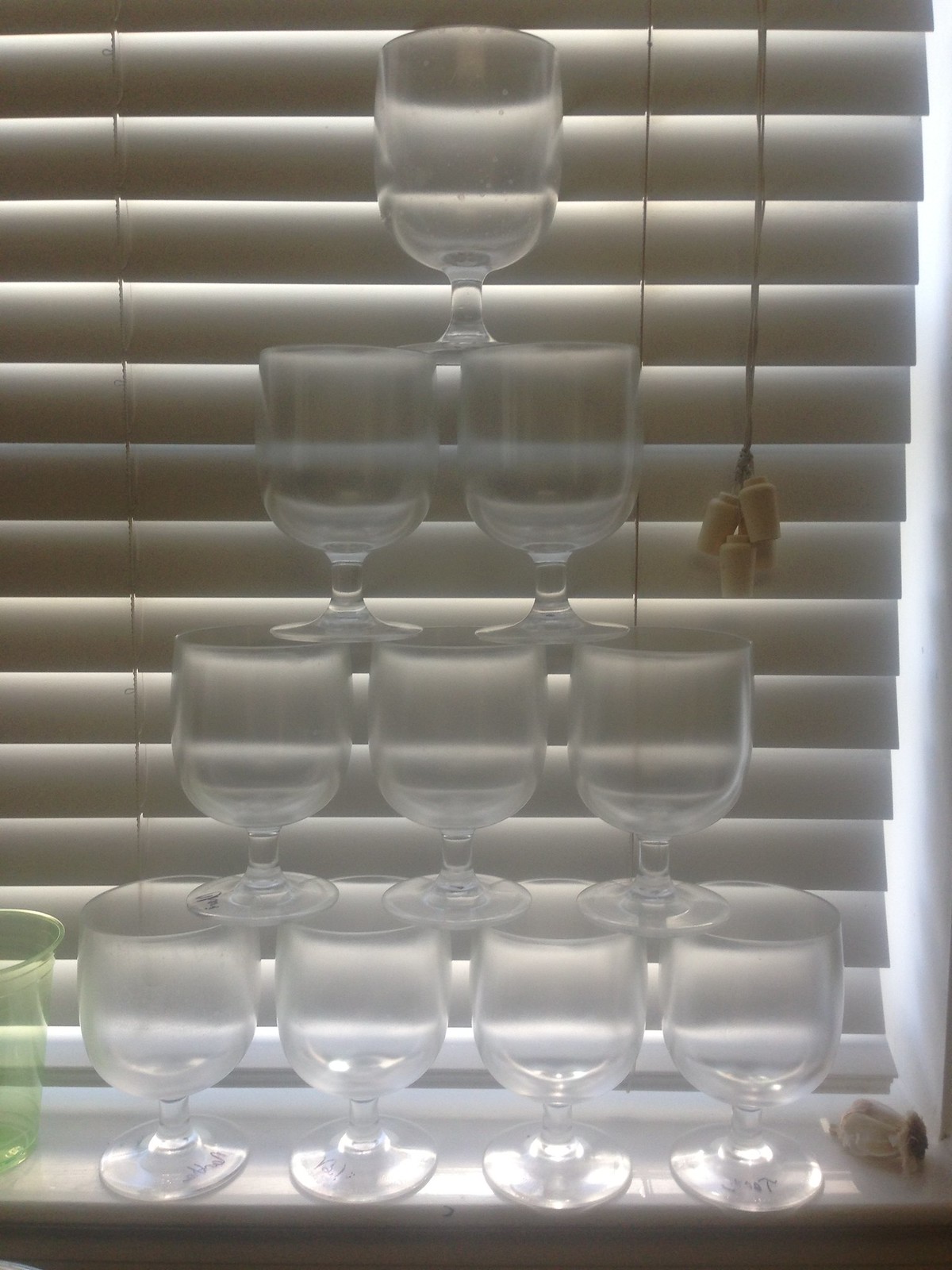In this photo, a white windowsill adorned with a closed white Venetian blind serves as the backdrop for an intricately stacked pyramid of clear, stemmed glasses, likely made of plastic rather than crystal. These glasses form a layered tower, with four glasses at the base, followed by progressively smaller upper layers of three, two, and finally, a single glass at the top, making a total of ten glasses. The glasses, which have short stems and straight, open tops, appear empty and lack the curvature typical of wine glasses, suggesting they are more likely water glasses. Hanging down from the upper right corner is a blind pole, featuring four cork-like weights at its end. On the far right edge of the windowsill sits a few cloves of garlic, while to the far left, a sliver of a greenish-yellow glass peeks into the frame.